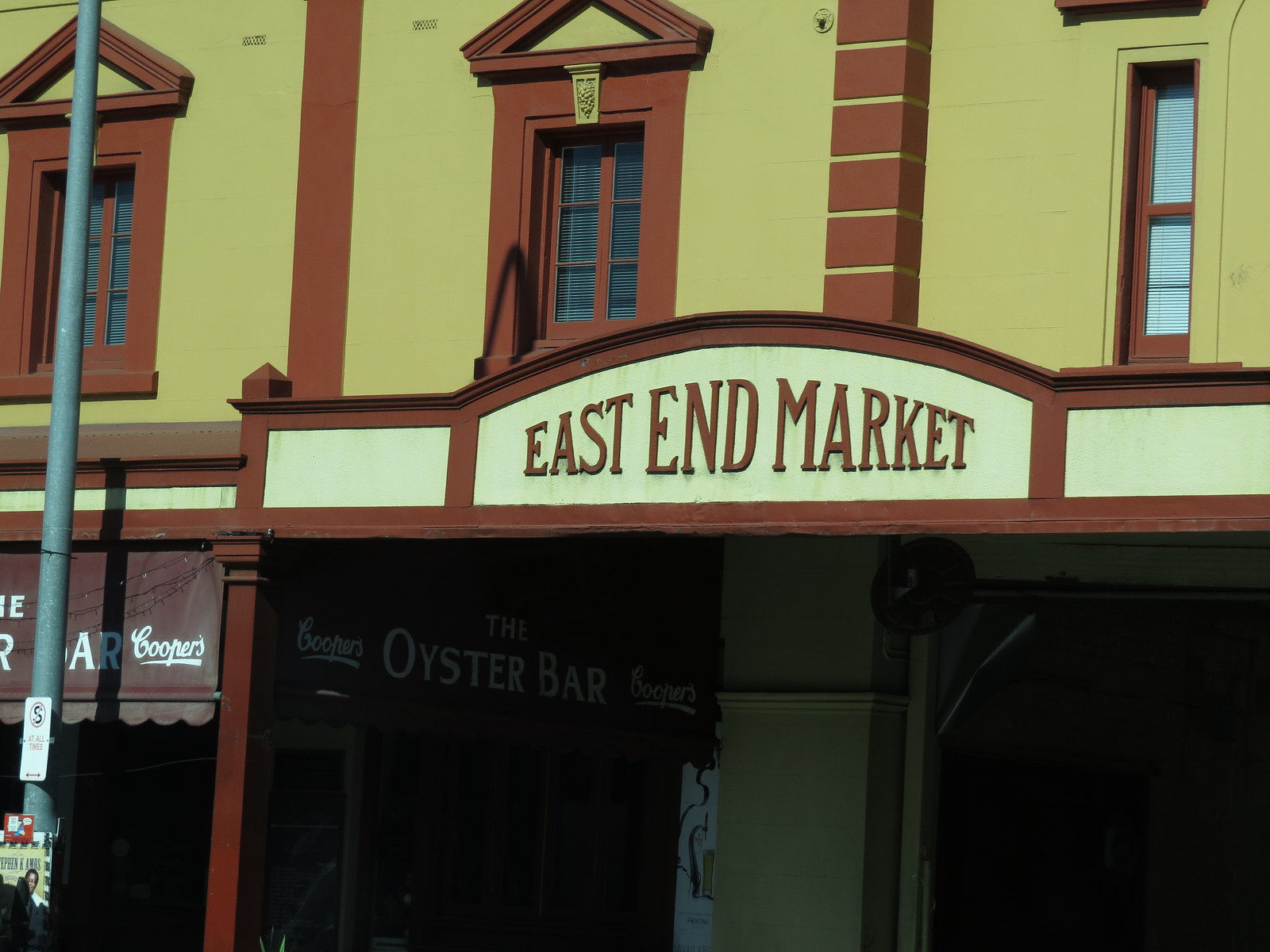This photograph captures the front façade of a charming two-story building. On the left side, there is a brown awning with white accents, partially obscured, but we can clearly see the side that mirrors the front design. The awning bears the name "The Oyster Bar" in bold white letters, and flanked around this name are the words "Coopers" on either side, hinting at a possible joint establishment.

The upper level of the building stands out with its warm yellow exterior and three windows, each framed in a contrasting rust color. The image is taken from a diagonal angle, giving us a partial view that adds an interesting dynamic to the shot. Prominently displayed on the yellow wall of the upper level is a rustic wooden sign. Matching the building's color palette, this sign blends in but is marked with large, rust-colored capitalized letters that read "EAST END MARKET."